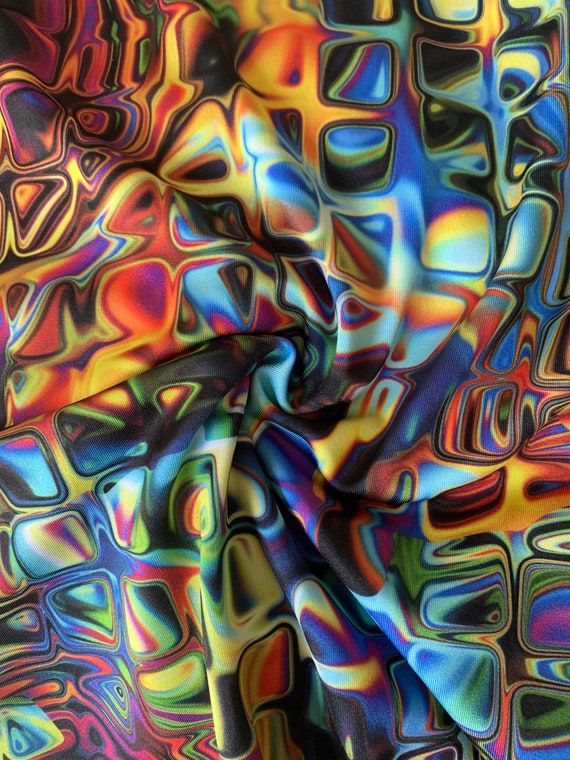This image displays an abstract, close-up view of a textile pattern rich in a vibrant, prismatic spectrum of colors, including reds, purples, oranges, blues, greens, and yellows. The fabric appears to have been picked up, twisted, and dropped, creating intricate folds and bends that warp the pattern in a dynamic, almost psychedelic manner reminiscent of thermal readings with hot and cold elements. The design features iridescent, one-inch cubes that are scattered across the fabric, lending an 80s or early 2000s feel to the overall aesthetic. The cubes transition from a reddish-orange on the left-hand side to a greenish hue in the middle, eventually blending into a bluish-purple towards the other side. The iridescent effect gives it a swirling, bubble-like quality, making the whole image feel like a timeless, groovy fabric pattern, possibly intended as a product photo highlighting the unique design.